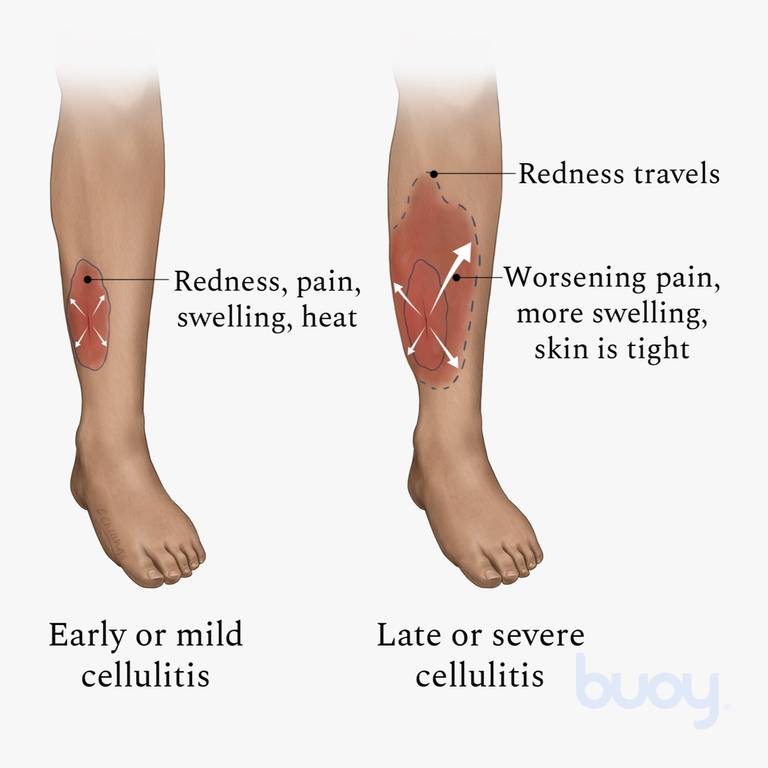This medical infographic, set against a light gray-green background, compares the progression of cellulitis in two stages. The image features two legs—from the knees down to the toes—with red patches indicating areas of infection. 

On the left, the leg shows an early or mild stage of cellulitis with a smaller, baseball-sized red patch located midway between the ankle and the knee on the inner shin. Four white arrows emanate from the center of this patch, symbolizing the spread of infection. A black label points to this area, highlighting symptoms such as redness, pain, swelling, and heat.

On the right, the image illustrates late or severe cellulitis. Here, the red patch has expanded considerably in size and has become more irregular in shape. Correspondingly, the white arrows are larger and more spread out. Labels point to this patch, indicating symptoms such as worsening pain, increased swelling, tight skin, and the spread of redness. There is a dotted outline around the larger red area to further emphasize the spread of the infection.

Both sections are clearly marked: "early or mild cellulitis" below the left leg and "late or severe cellulitis" below the right leg. The infographic bears a watermark in the bottom right corner that reads "buoy."